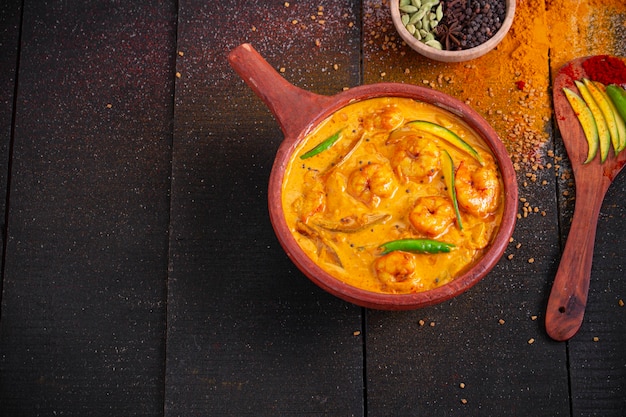The photograph depicts a close-up scene featuring a rich, rustic setting on a dark brown, wooden slatted table. At the center is a reddish-brown wooden bowl with a handle, containing a vibrant orange curry sauce brimming with shrimp and chunky bits, complemented by slices of avocado and green chili pepper. Adjacent to the bowl is a wooden serving spoon holding sliced avocado sprinkled with paprika. Adding to the visual feast, a small ramekin filled with various spices, including anise stars and cloves, sits nearby. The table itself is scattered with additional spice powders, creating a vivid contrast with the dark, rustic backdrop, enhancing the bright, appetizing colors of the curry and the garnishes.